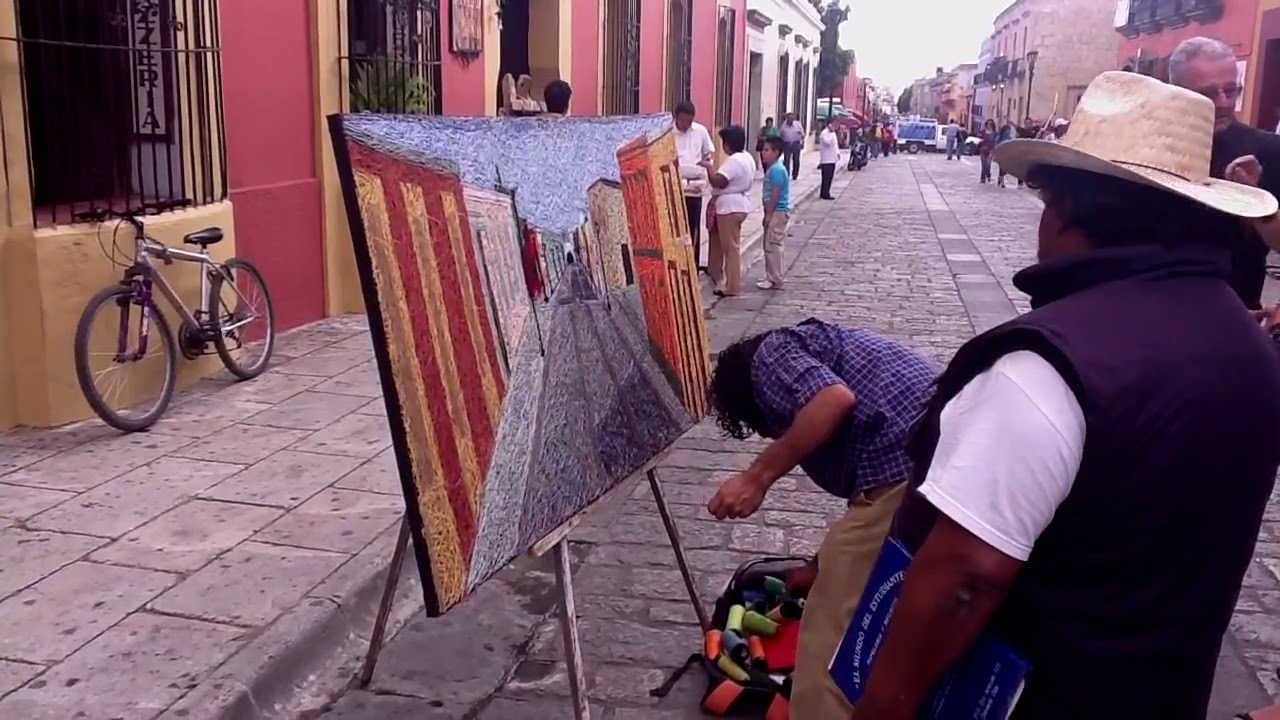The photograph captures a vibrant street scene featuring a pair of street artists. Dominating the right side of the image is an easel holding a painting that depicts the very street where the action unfolds. This self-referential artwork shows buildings with red, yellow, and white facades, mirroring the real architectural hues around them. One artist, dressed in khaki pants and a short-sleeved blue shirt, is bent over, rummaging through a bag. His companion, a man in a purple vest over a white t-shirt, stands straight with a book in hand, watching attentively while wearing a tan hat. 

The street, lined with light-colored brick paving, is bustling with pedestrians, some milling about while others engage in their own activities. A bicycle is parked behind the easel, its wheel visible on the left side of the picture. The scene is set against the backdrop of similarly colored buildings—yellow and a pinkish hue—with people scattered in the distance. The daylight enhances a spectrum of colors visible in the photo, including shades of orange, yellow, light blue, brown, teal, and tan, contributing to the lively urban atmosphere.